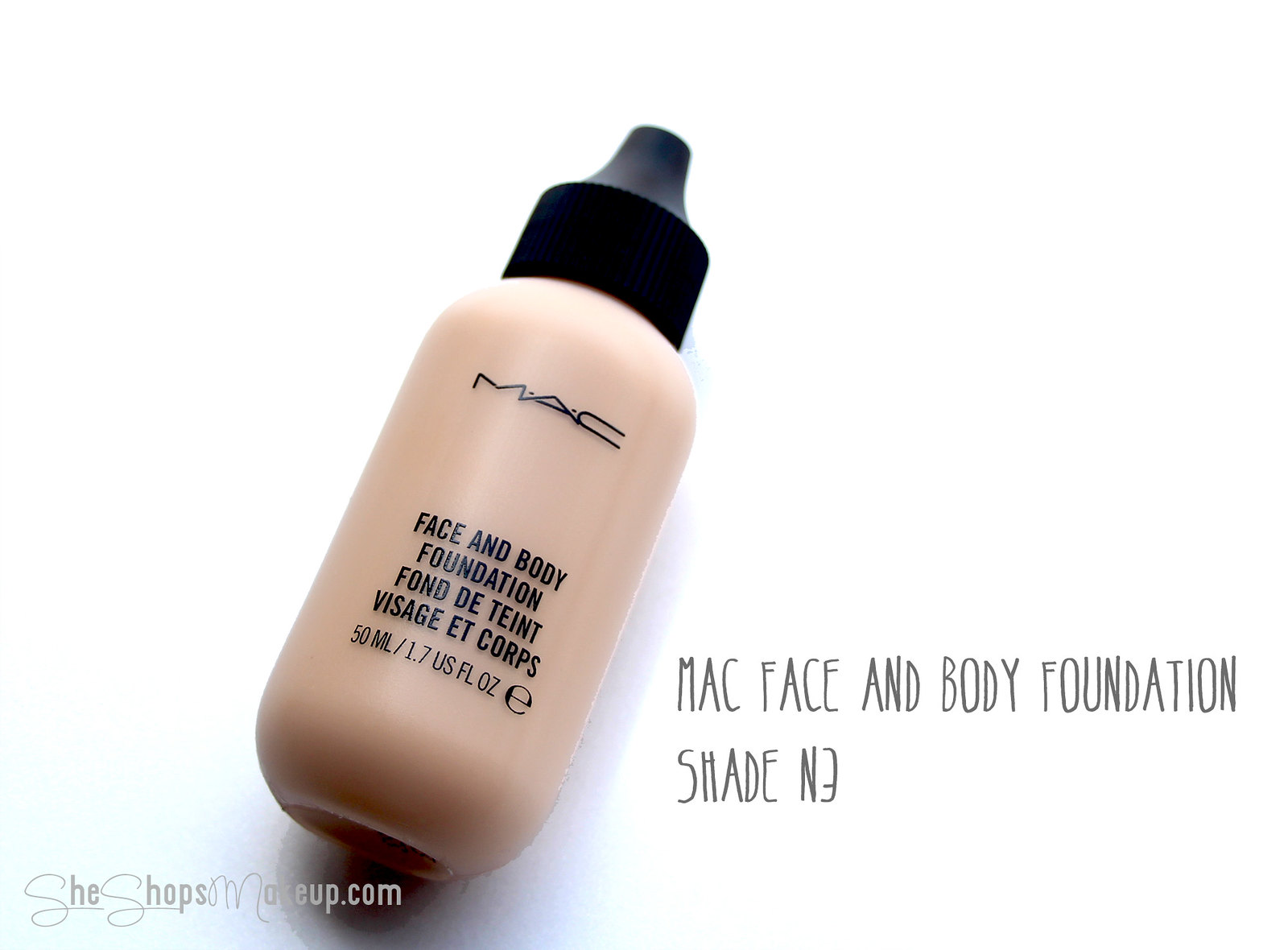This advertisement showcases a MAC Face and Body Foundation in a shade between dark brown and creamy tan, specifically labeled as N3 with a reversed "E." The product is presented in a close-up photograph against a bright, clean white background. The bottle, holding 1.7 fluid ounces of foundation, is laid on its side, casting a subtle shadow to the right from the viewer's perspective, which would be the left side if oriented from the bottle's viewpoint. The foundation comes in a small cylindrical bottle featuring a black cap and the iconic MAC branding in simple black capital letters. Beside the bottle is the product name "MAC Face and Body Foundation" in gray text. Below the bottle, the URL "sheshopsmakeup.com" is provided, guiding consumers to purchase the product.